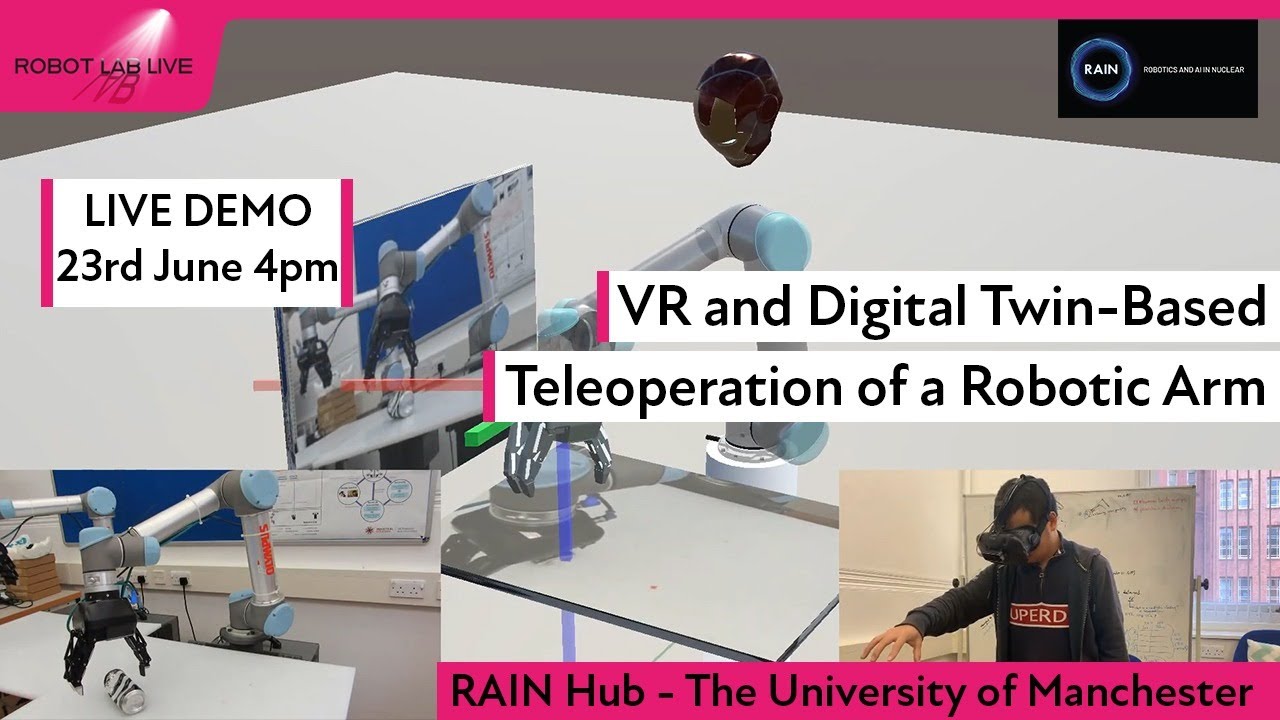This is a detailed flyer for a live demonstration happening on the 23rd of June at 4:00 PM, titled "Robot Lab Live". The flyer is in landscape format with a pink line at both the top and bottom. At the top, in black font, the words "Robot Lab Live" are prominently displayed with a spotlight shining on the word "Lab", reflecting below. In the upper right-hand corner, the logo "RAIN" within a blue circle is set against a black background, alongside the words "Robotics and AI in Nuclear".

The flyer features three images: one of a robotic arm performing tasks such as picking up a can, another of a man wearing a virtual reality headset with a whiteboard in the background, and a final image of another piece of robotic machinery. Below these images, centered at the bottom, the text reads "RAIN Hub / the University of Manchester". Additionally, there is a white text block in the middle of the flyer that highlights the main event: "VR and Digital Twin Based Teleoperation of a Robotic Arm". Off to the left, in a smaller white box with a pink border, it indicates "Live Demo, 23rd of June, 4 PM" in black letters.